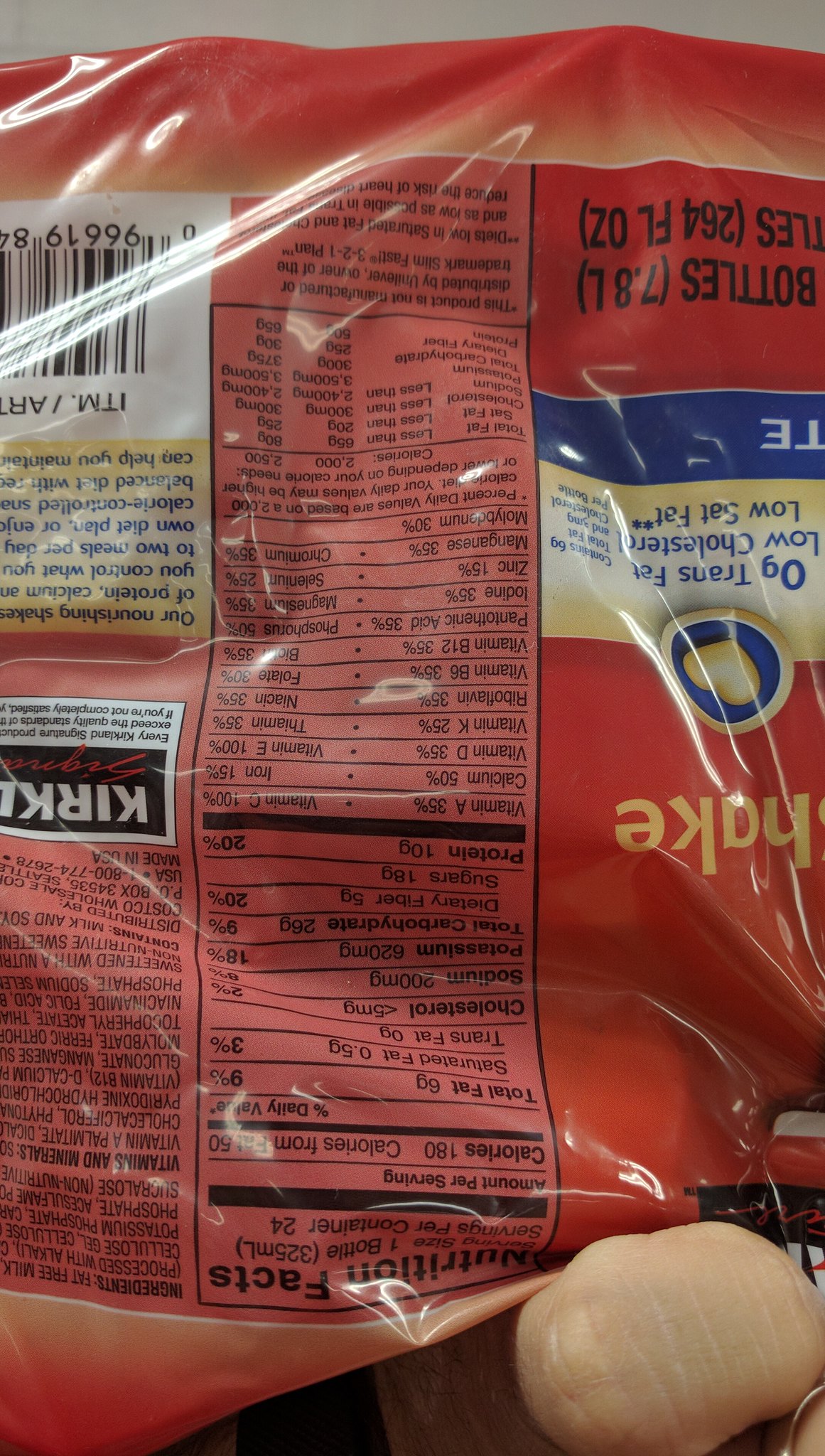A high-resolution image features a very shiny package that appears to have been inadvertently dropped upside down. Due to the orientation, the lettering on the package is difficult to read. From the visible text and design, it is clear that this is the back side of the package, evidenced by the presence of nutritional facts and a list of ingredients. The background color of the package is predominantly black. On the left-hand side of the package, partially obscured text spells out "K-I-R-K-L." The right-hand side displays another partially visible text in bold yellow letters spelling out "H-A-K-E." In front of the package, prominently displayed, is a fresh, raw potato positioned next to the package, underscoring the freshness and natural ingredients associated with the product. The entire scene is meticulously detailed, capturing the shiny texture of the package and the earthy look of the potato.